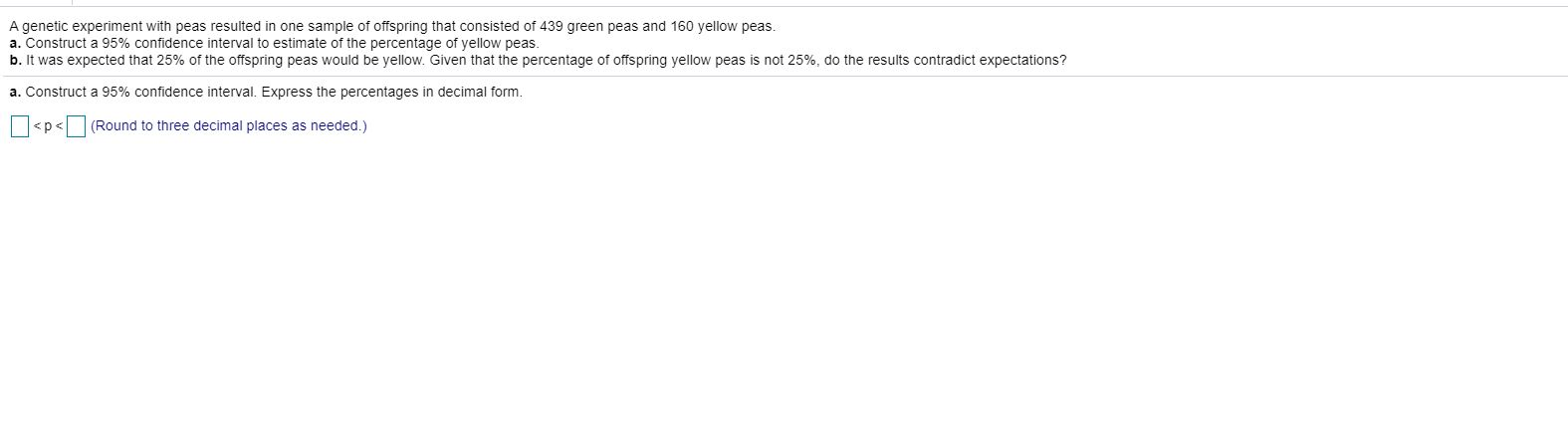This screenshot features a small and somewhat challenging-to-read segment of text, primarily composed of numeric data and instructions. The text explains a genetic experiment involving peas, with the sample producing 439 green peas and 100 yellow peas. It instructs to use a 95% confidence interval to estimate the percentage of yellow peas and assess whether the experimentally observed percentage aligns with the expected 25% yellow peas. Below the main text, there are prompts for input, including a field to express the confidence interval in decimal form and another field to calculate and enter the probability (P), both requiring up to three decimal places.